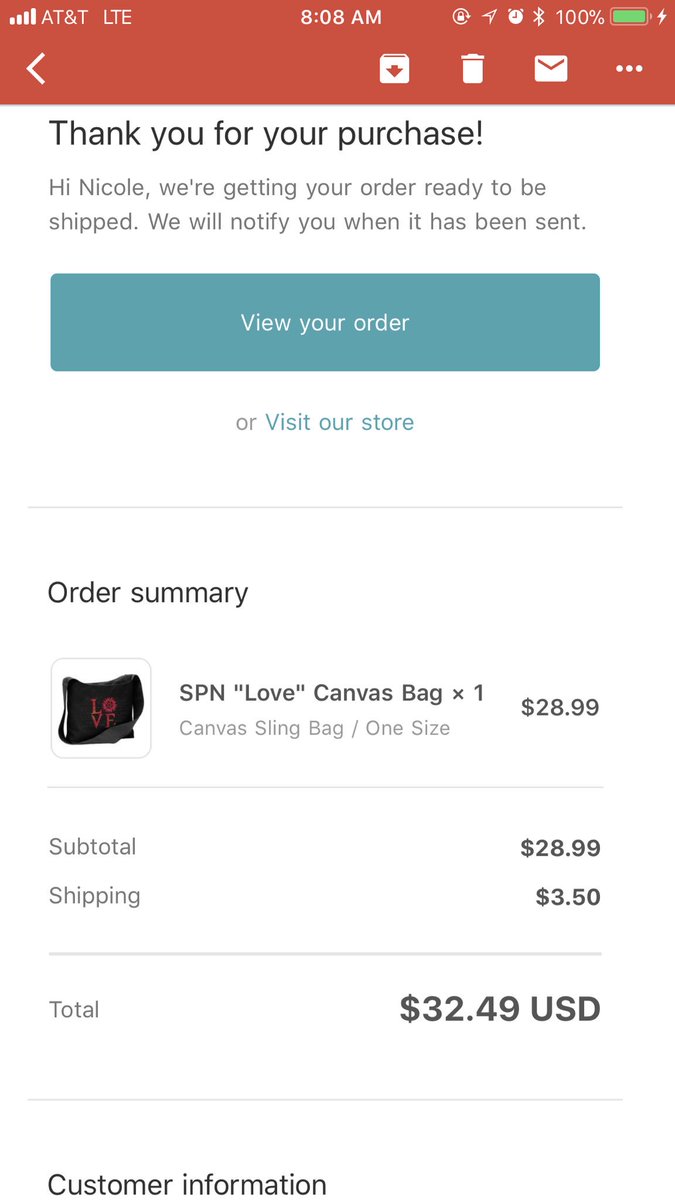Here is a cleaned-up and detailed caption for the image:

---

This image captures a screenshot taken from a mobile device. At the top of the screenshot, there are the usual mobile device icons indicating network connection, the current time, Bluetooth connectivity, and battery status. Below these icons, the email application interface is displayed. The top section of the app features a red rectangular box with several icons inside it, including options to archive emails, delete emails, create a new email, and a menu represented by three dots for additional options.

The email displayed in this screenshot is a purchase receipt. The subject line of the email reads, "Thank you for your purchase." Within the email, there is a prominent blue box that can be tapped to view the order details, and there is also a hyperlink to visit the store's website.

The email contains an order summary featuring a small thumbnail image of a black canvas bag, labeled "SPN 'Love' Canvas Bag" with a quantity of one. The price of the bag is listed as $28.99. The email also details additional charges, including a shipping fee of $3.50, bringing the total cost of the order to $32.49.